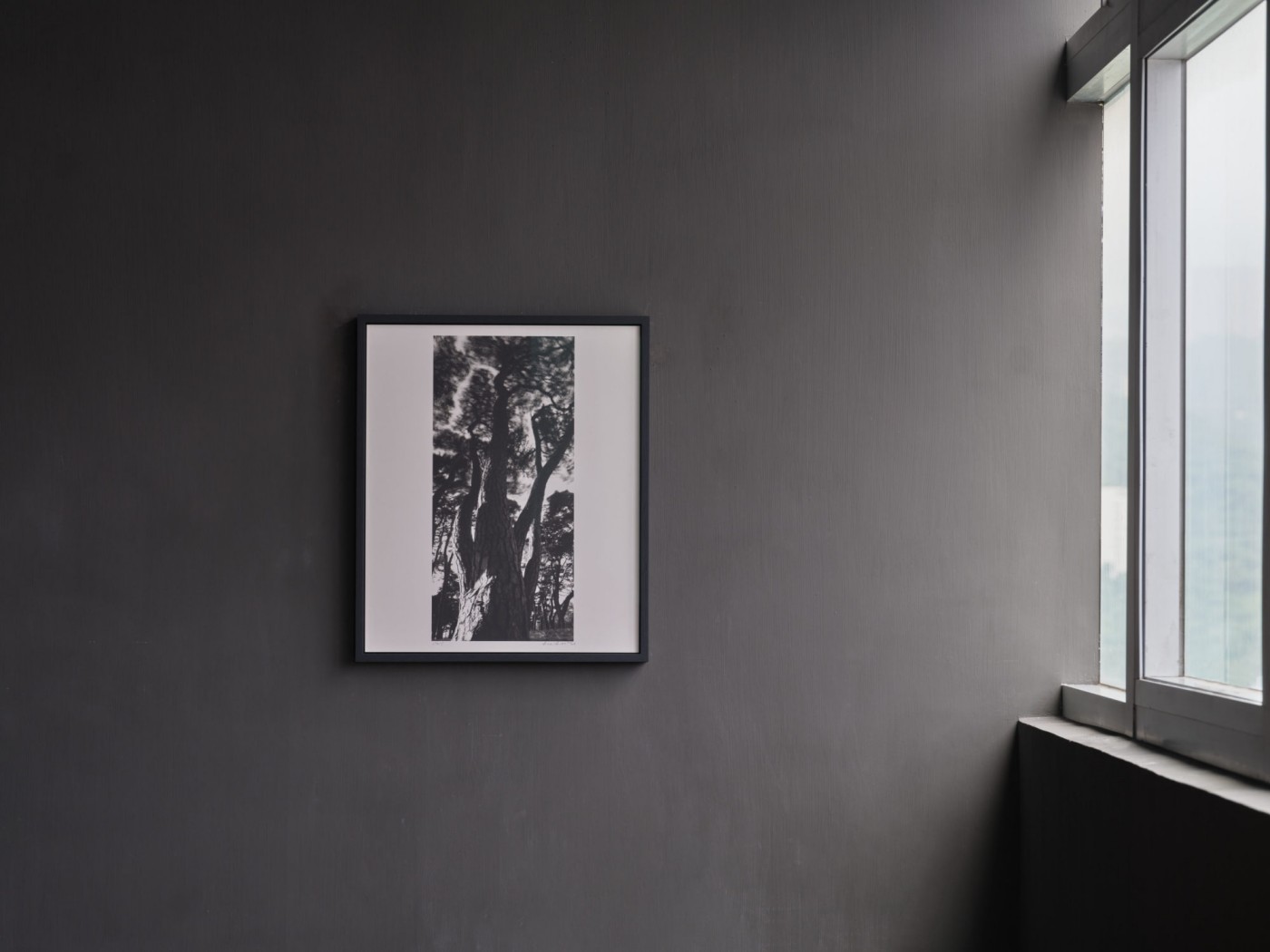This image features a predominantly dark gray wall with a window on the right side. The window spans from the top right corner down to nearly the bottom right corner, appearing hazy and slightly obscured. While initially resembling a black-and-white photograph, a faint bluish hue in the sky outside the window suggests that the room itself is simply monochromatic. Centered on the wall is a framed print; the frame is black, paired with a very light gray mat. The print within is a narrow piece of modern abstract art, composed of various shades of black, featuring an array of splotches, lines, and squiggles, devoid of any direct reference to reality.